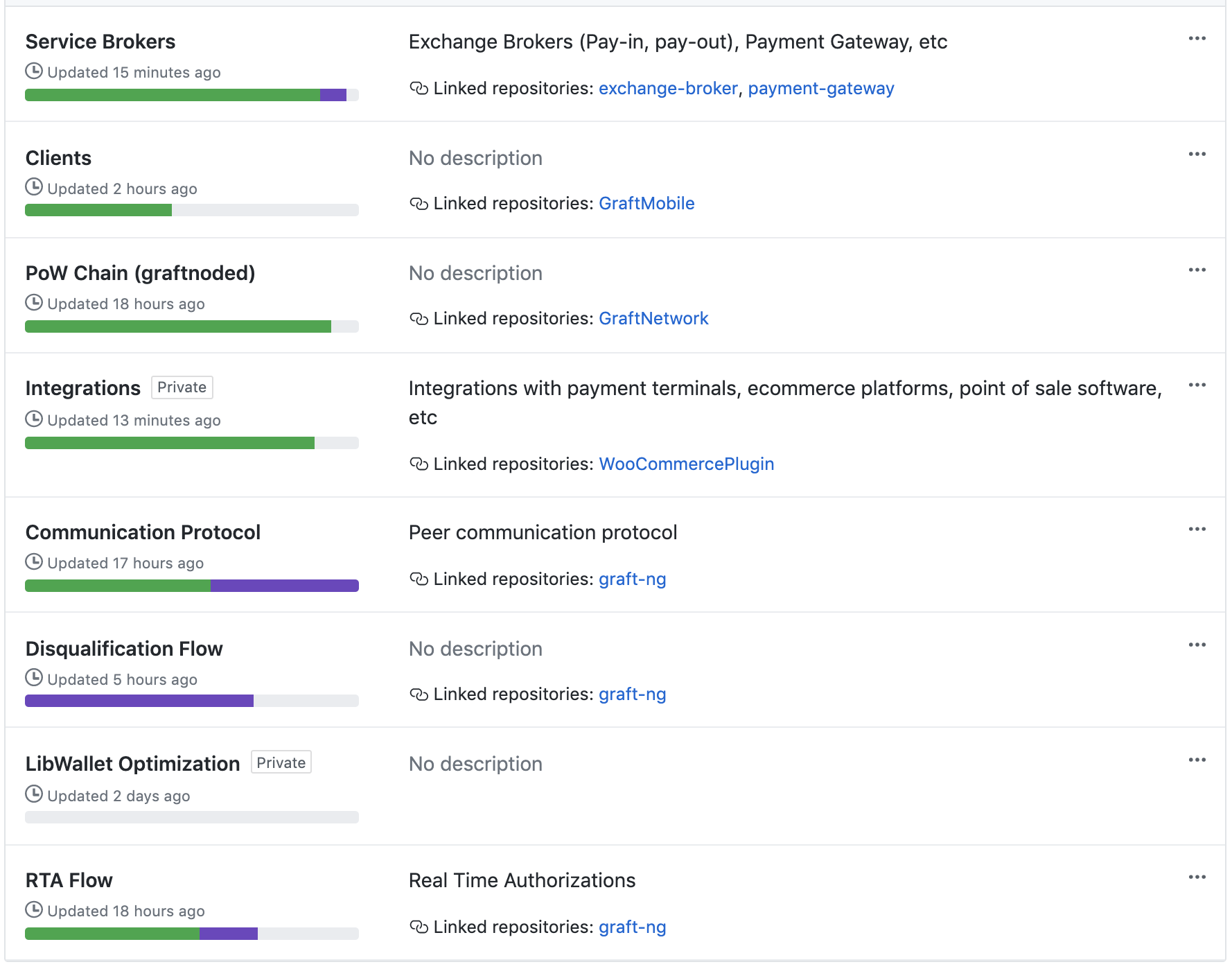Here is a detailed and cleaned-up caption for the image you described:

---

Screenshot of a web application dashboard featuring a two-column layout against a white background with a thin light gray border surrounding it. The dashboard is organized into seven rows, each with specific content and status indicators.

- **Header Area:**
  - At the top, there's a very thin light gray bar running horizontally across the interface, slightly darker below it, acting as a header separator.

- **First Row:**
  - **Left Column:**
    - Bold black text reads "Service Brokers".
    - Below, a small clock icon indicates "Updated 15 minutes ago".
    - A progress bar shows near-full capacity, primarily green with a small segment of blue and light gray indicating the incomplete portion.
  - **Right Column:**
    - Text reads "Exchange Brokers, Pay In, Pay Out, Payment Gateway", followed by clickable links "Linked Repositories: exchange-broker, payment gateway".
    - A three-dot menu icon for additional options.

- **Second Row:**
  - **Left Column:**
    - Bold text reads "Clients".
    - A clock icon notes "Updated 2 hours ago".
    - The progress bar, filled about 40% in green, with the remainder in light gray.
  - **Right Column:**
    - Text "No description" on the first line.
    - Below, clickable links "Linked Repositories: craft mobile".
    - A three-dot menu icon.

- **Third Row:**
  - **Left Column:**
    - Bold text reads "Pow Chain (Graft Noted)".
    - A clock icon states "Updated 18 hours ago".
    - The bar is nearly full (90-95% green), only a small part in light gray.
  - **Right Column:**
    - "No description" followed by clickable links "Linked Repositories: graph network".
    - A three-dot menu icon.

- **Fourth Row:**
  - **Left Column:**
    - Bold text "Integrations", with a small private label badge.
    - A clock icon shows "Updated 13 minutes ago".
    - The progress bar is about 85-90% green, with a bit in light gray.
  - **Right Column:**
    - Text "Integrations with payment terminals, e-commerce platforms, point of sale software, etc."
    - Below are clickable links "Linked Repositories: WooCommerce plugin".
    - A three-dot menu icon.

- **Fifth to Seventh Rows:**
  - **Multiple Entries with Diverse Content:**
    - One entry titled "Disqualification Flow" contains a progress bar roughly 70% blue, the rest light gray.
    - Other rows may be empty or similarly structured with a header, update time, description, progress bar, and a three-dot menu icon.

In all rows, consistent formatting includes a bold title, an update timestamp, progress bars with varied levels, descriptions, linked repositories, and menu icons.